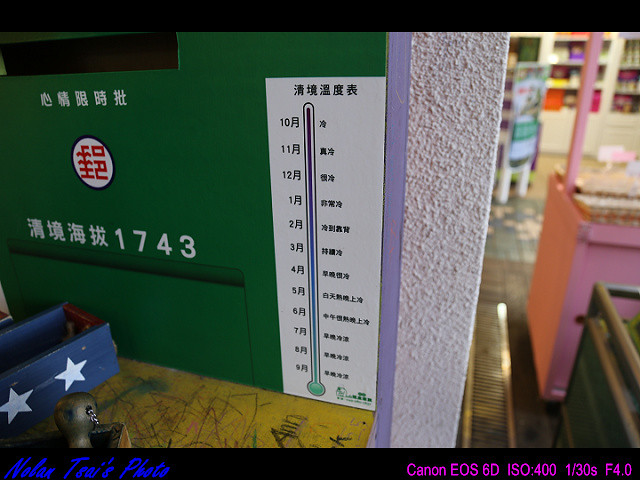This photograph features a richly detailed scene. On the bottom left, blue text reads, "Nolan's Illegible Photo," while to the right, pink text provides camera details: "Canon EOS 6D, ISO 400, 1/30th, f/4.0."

The focal point of the image is a dark green wall adorned with Asian script and the number "1743." Attached to this wall is a thermometer, also displaying Asian writing. In the foreground, there is a wooden table, its surface marked by colorful scribbles and writings.

Adjacent to the table is a navy blue wooden box, embellished with white stars. At the center of the photograph, a stucco wall painted with a lavender stripe down the middle adds a contrasting texture. To the right of this wall, part of what appears to be a shop or a café becomes visible, possibly featuring various tables and items that suggest a communal or commercial space.